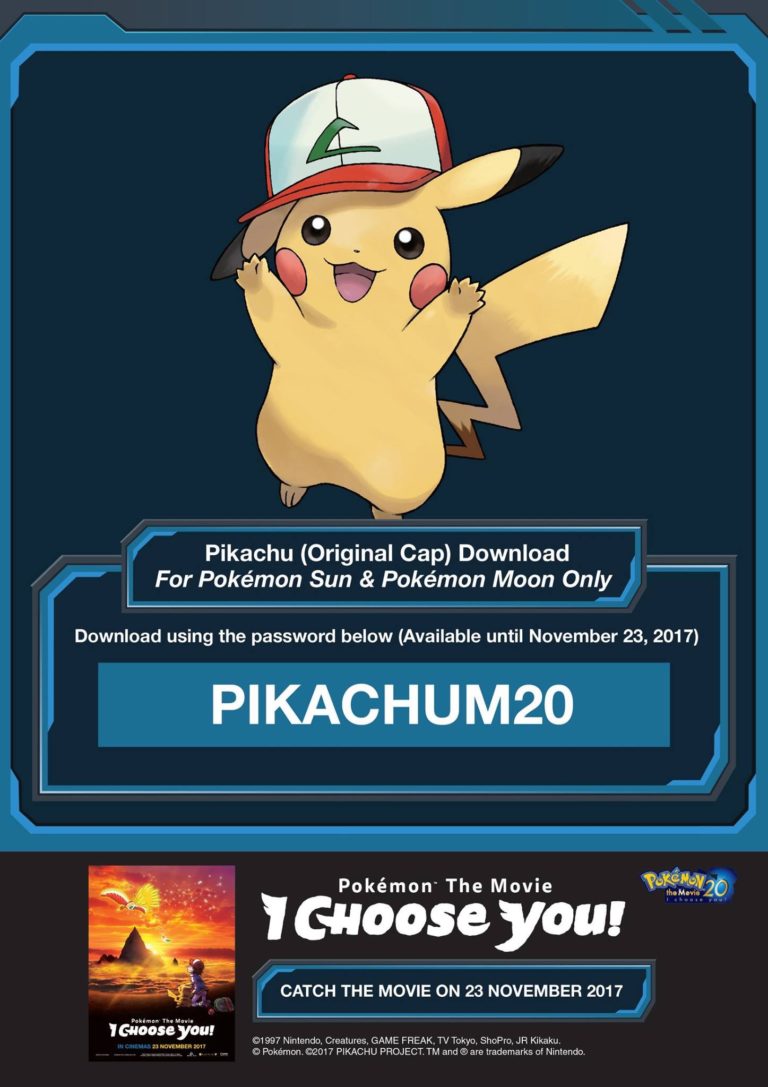This rectangular image features a black background and prominently displays a joyous Pikachu positioned at the top center, wearing a distinct red and white cap adorned with a triangular logo. Below Pikachu, text reads: "Pikachu Original Cap. Download for Pokémon Sun and Pokémon Moon only. Download using the password below, available until November 23, 2017." The specified password is displayed as "P-I-K-A-C-H-U-M-2-0".

In the lower segment of the image, promotional text states, "Pokémon the Movie: I Choose You. Catch the movie on November 23, 2017." To the left, there is a poster for the movie depicting a boy gazing into what appears to be an ocean scene, with a barely recognizable Pikachu by his side. The backdrop is a rich, red sky, and the words "I Choose You" are clearly visible.